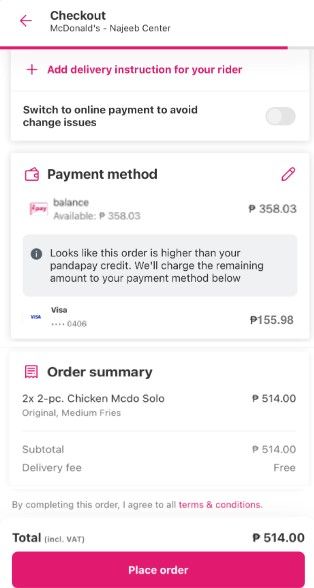The image displays a checkout screen from McDonald's located at Najeeb Center. At the top of the screen, the phrase "Check Out" is prominently displayed. Below it, there are delivery instructions encouraging users to switch to online payments to avoid issues with change. This particular order has a balance of $358.03 in what appears to be an unfamiliar currency symbol. 

The order summary includes:
- 2 x 2-piece Chicken McDo (solo)
- Original Medium Fries

The subtotal for the order is $514.00, and the delivery fee is waived. The total amount, including VAT, remains $514.00. The screen also notes that the available Panda Pay credit covers part of the order but falls short, necessitating a charge to a Visa card (ending in 0406) for the remaining amount of $155.98.

The user is required to agree to the terms and conditions by completing the order, which can be done by pressing a large red "Order" button at the bottom of the screen. The interface features a white background with black and red fonts.